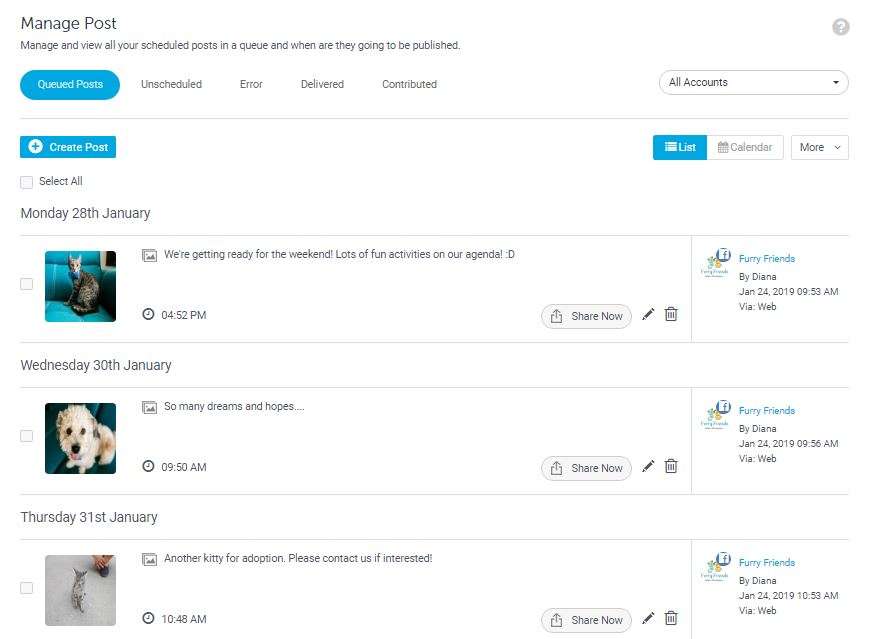This image depicts a detailed screenshot of a social media management interface for scheduling posts. At the top of the screen, bold black text reads "Manage Post". Below that is an explanatory line in smaller print: "Manage and view all your scheduled posts in a queue and when they are going to be published."

Prominently featured in cyan blue is a pill-shaped button labeled "Queued Posts". Surrounding this button on a white background are the words "Unscheduled, Error, Delivered, Contributed" in black print, each starting with a capital letter.

To the right of these options is a drop-down menu labeled "All Accounts". Beneath this line is another banner in a medium blue color, which contains a circular icon with a plus sign and the text "Create Post" in cyan font. Opposite this, there are options to switch the view: a blue square labeled "List", a white square labeled "Calendar", and a drop-down menu labeled "More". There is also a small square checkbox accompanied by the text "Select All".

The section below this interface displays scheduled posts by date. 

- The first post is scheduled for Monday, January 28th, and features an image of a cat with the caption: "We're getting ready for the weekend. Lots of fun activities on our agenda." Options to share, edit, or delete this post are provided. It is credited to "Furry Friends by Diana".
  
- The second post scheduled for Wednesday, January 30th showcases a photo of a dog accompanied by the caption: "So many dreams and hopes." Similar options to share, edit, or delete this post are available, also credited to "Furry Friends by Diana".

- The final post scheduled for Thursday, January 31st features another cat with the caption: "Another kitty for adoption. Please contact us if interested." As with the other posts, users can choose to share, edit, or delete this post, and it is credited to "Furry Friends by Diana".

This comprehensive schedule view enables users to manage and organize their social media content efficiently.